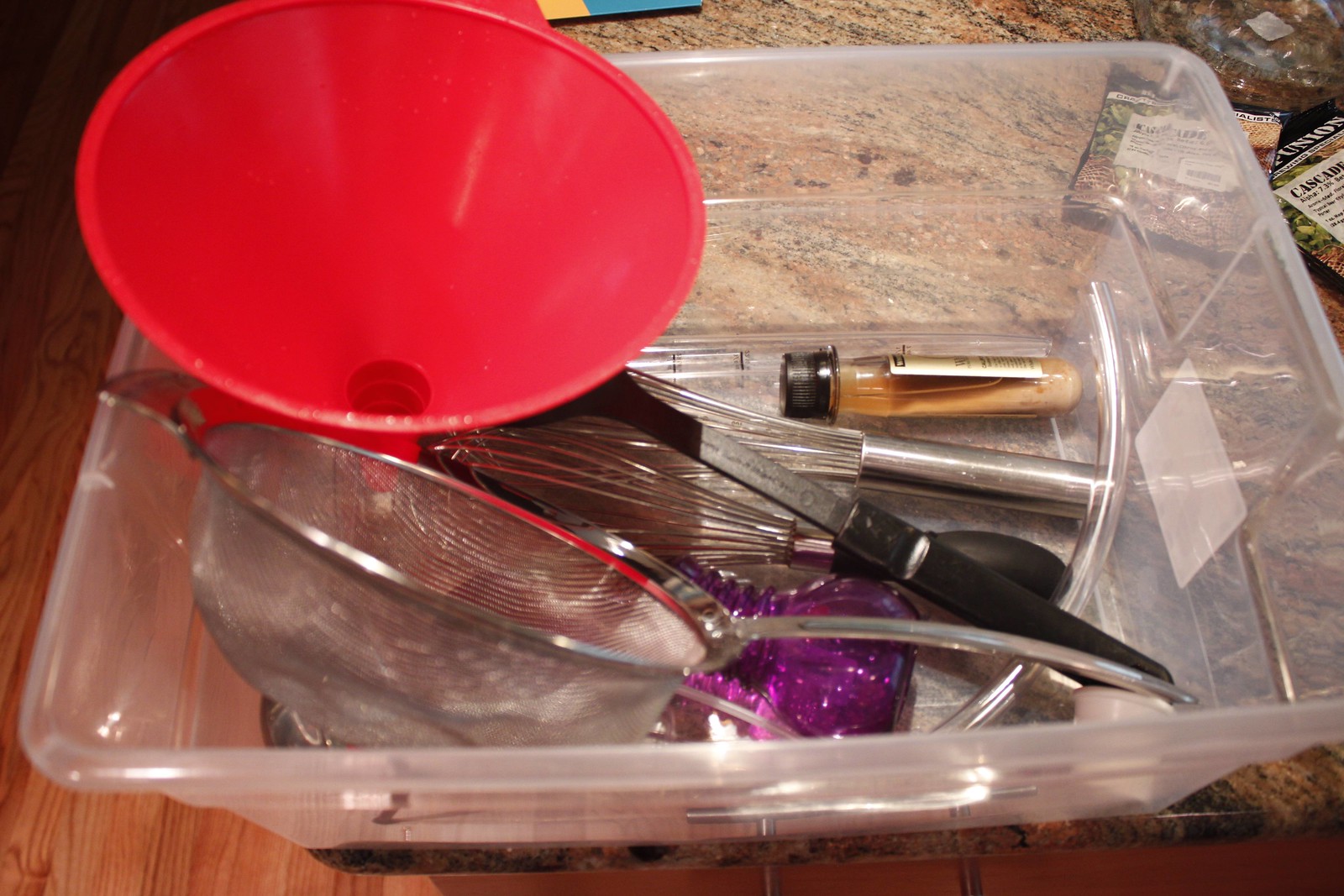A well-worn brown work table, showing signs of frequent use especially at the front, is scattered with various objects. The surface features several black spots contrasting against the brown wood. At the center, a sheet of paper adorned with blue and yellow hues lies partially obscured. To the side, a small glass ashtray is positioned near two plastic packets, each with a distinctive black top and a white label with black writing. Dominating the scene is a large white plastic tub, centrally placed, containing a red plastic funnel and a metal strainer suitable for sifting flour or straining liquids. Inside the tub, there are two whisks, a metal one and another possibly of a different material, along with a small bottle filled with a brownish-white fluid, topped with a black cap and a gold label. A purple bottle, potentially used as a vase or flower container, sits lower down the scene, with what appears to be a knife protruding from its top.